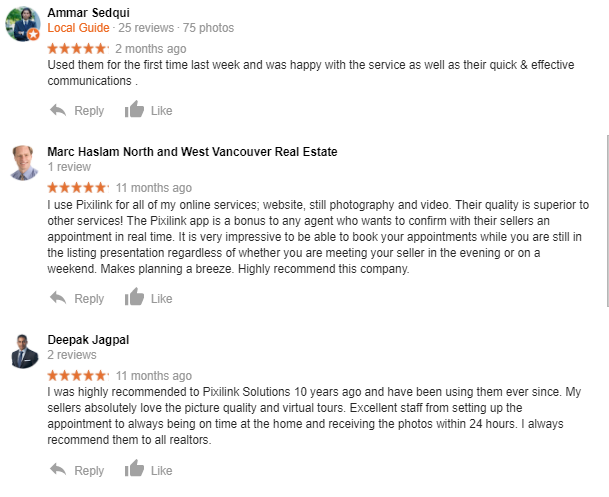Underneath the caption, with intricate details, I have restructured and refined it to create a cohesive and comprehensive descriptive caption:

---

**Image Caption:**

The image depicts a forum-like comment section featuring reviews and testimonials for a service provider. Starting from the top, user "Amar Saeed-Quain" has posted a comment. His profile picture is shown in a circular frame beside his name, where he is seen wearing a blue blazer and a tie. Underneath his name, there is an orange badge indicating "Local Guide," followed by gray text showing "25 reviews, 75 photos." Additionally, an orange five-star rating is prominently displayed, along with a timestamp reading "2 months ago" in gray text. His review states: "Used them for the first time last week and was happy with the service as well as their quick and effective communications." Below his comment, there are "Reply" and "Like" buttons.

Following Amar's review, there is a comment from "Mark Haslam," whose title reads "North and West Vancouver Real Estate." Mark has left one review and rated the service five stars. His review dates back "11 months ago." Mark's detailed testimonial praises Pixlink: "I use Pixlink for all my online services, including website, still photography, and video. Their quality is superior to other services. The Pixlink app is a bonus to any agent who wants to confirm appointments with their sellers in real-time. It is very impressive to be able to book your appointments while you're still in the listing presentation. Regardless of whether you are meeting your seller in the evening or on a weekend, it makes planning a breeze. Highly recommend this company." Similar to the previous comment, "Reply" and "Like" buttons are available.

The final comment is from "Deepak Jagpal," who has left two reviews and rated the service five stars as well, dating back "11 months ago." Deepak extols the company's services: "I was highly recommended to use Pixlink solutions 10 years ago and have been using them ever since. My sellers absolutely love the picture quality and virtual tours. Excellent staff, from setting up the appointment to always being on time at the home and receiving the photos within 24 hours. I always recommend them to all realtors." At the bottom of his comment, "Reply" and "Like" buttons are also present.

Each user's feedback highlights various positive aspects of Pixlink's services, underscoring their satisfaction and recommendations.